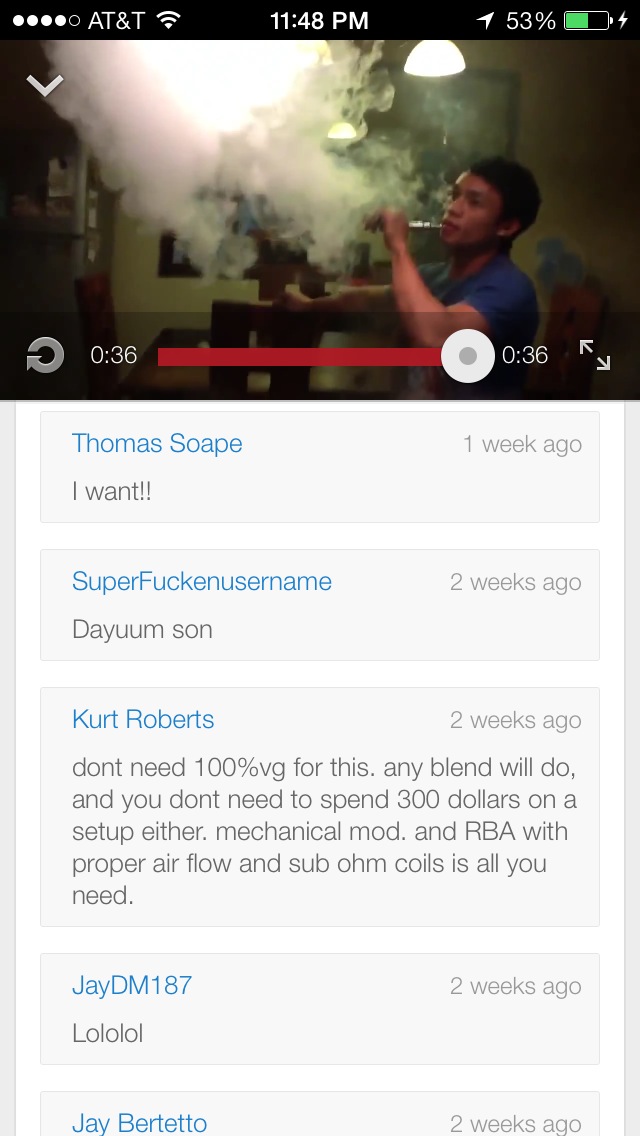The image showcases a detailed screenshot from a phone screen showing a video at its end. The device, using AT&T as the carrier, displays the time as 11:48 p.m. with a 53% battery level. The video depicts a young Asian boy in a short-sleeved blue shirt vaping, producing a large plume of white smoke visible in front of him. The video duration is 36 seconds, with the progress bar indicating it is fully played, and there is an option to replay or expand the video for full-screen viewing.

Below the video, various comments are visible:
- Thomas Soap commented, "I want" one week ago.
- User "Super Fucking Username" reacted with, "damn son" two weeks ago.
- Kurt Roberts shared, "Don’t need 100% VG for this. Any blend will do, and you don't need to spend $300 on the setup either. Mechanical mod and RBA with proper airflow and sub ohm coils is all you need," also two weeks ago.
- JDM 187 added, "LOL LOL LOL" two weeks ago.

This capture not only provides a snapshot of the moment in the video but also a glimpse into the community engagement surrounding it.